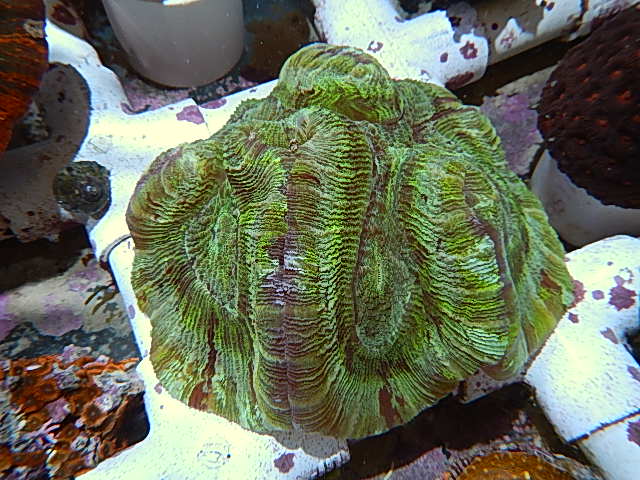In this square drawing, the centerpiece is an irregularly shaped, round object with a circular notch at the top. The object is predominantly green with shades of brown and gray, featuring a bumpy texture that resembles snake skin or perhaps a head of cabbage. Surrounding this central figure are white pipes in each corner, some with rust or peeling paint revealing red or reddish-brown underneath. The upper left corner features a dark gray item reminiscent of the bottom half of a computer mouse. In the upper right corner, there's a half-circular, medium brown object with small holes, possibly crocheted, showing red hues peeking through. Additionally, the background includes various mysterious items like a striped cloth on the left and a pink and red item with floral patterns in the bottom left corner.